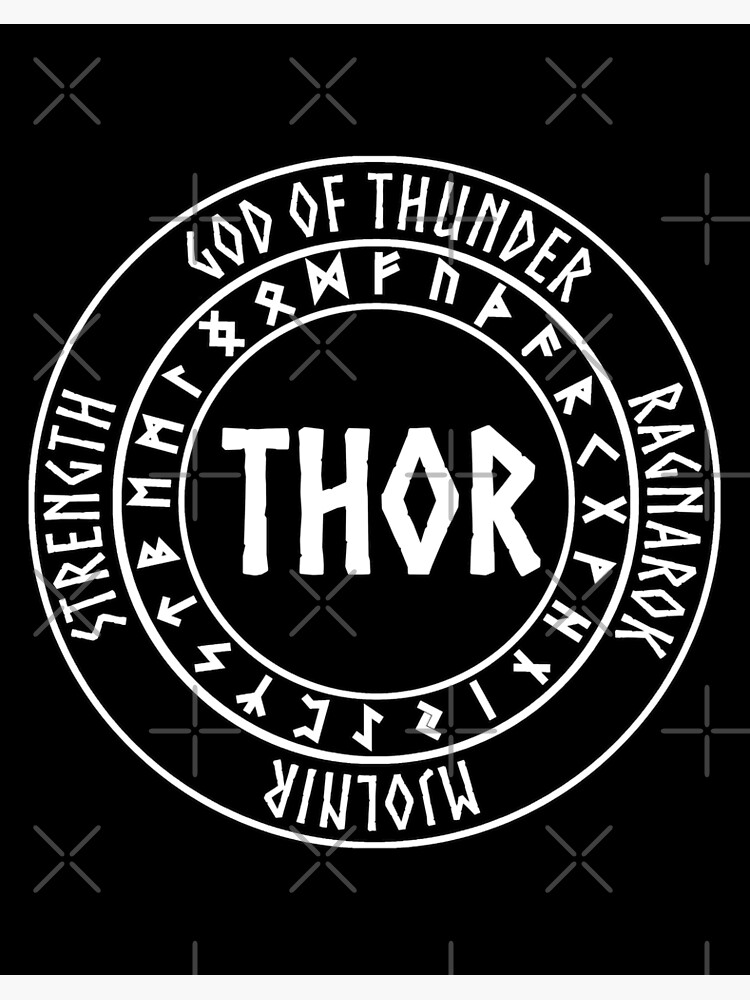The image showcases a logo design set against a black background, with the text "WarlordApparel" positioned in white in the bottom right corner. The main design features a series of concentric circles in black and white. The outermost circle is inscribed with the phrases "God of Thunder" at the top, "Ragnarok" on the right, "Strength" on the left, and "Mjolnir" at the bottom (though one word is upside down and could be less visible). Moving inward, the next ring contains a collection of symbols or hieroglyphs that appear to be Norse runes. At the very center of the logo, the name "Thor" is prominently displayed in bold white letters. This intricate and monochromatic design likely represents themes from Norse mythology and appears to be the creation of the brand Warlord Apparel.